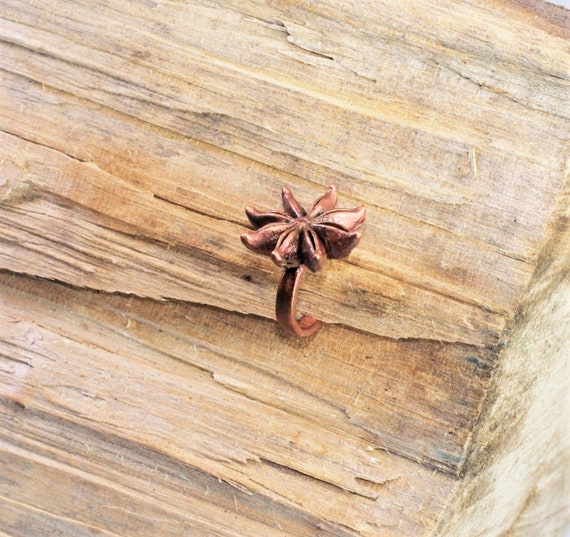This image features a close-up view of a piece of wood, which appears jagged, uneven, and splintered, especially on the bottom right. The wood shows a horizontal grain pattern, transitioning from light brown to darker brown with some blackened edges. In the center of this wooden surface sits a distinctive copper-colored ring adorned with a flower-like ornament on top. The flower-like figure is reminiscent of a star anise, consisting of seven petals and appearing to grow out of a brown stem or metallic hook that is partially embedded into the wood. The overall aesthetic of the photograph is subtle, with even lighting that harmonizes the earthy tones of the wood and the copper ring, drawing subtle attention to the intricate design of the central object.